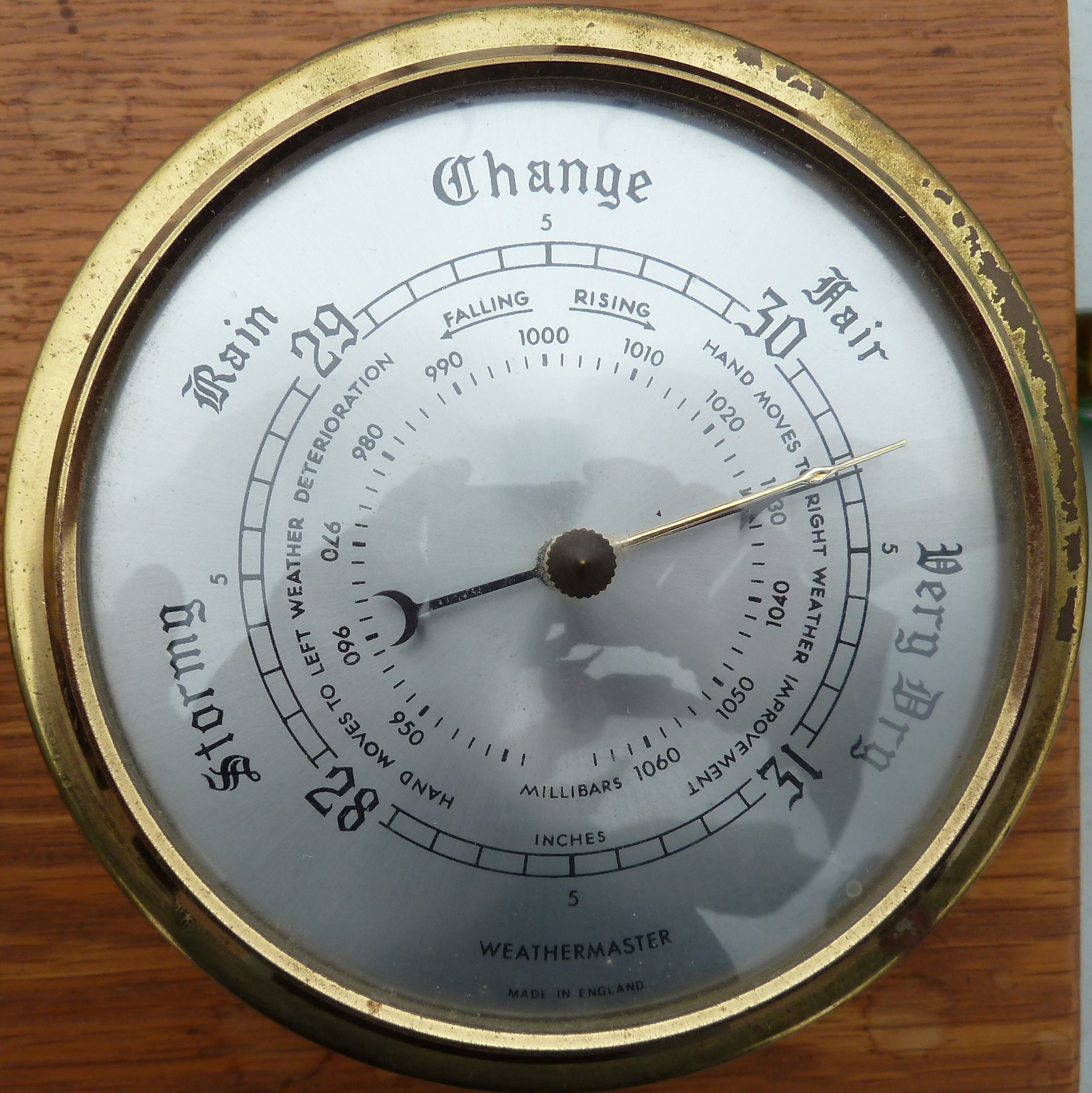The image depicts a square photo of a round Weathermaster barometer, prominently framed in a chipped gold outline and placed atop a light brown wooden surface. The circular barometer almost touches the photo's edges and is encased in a domed glass cover. The interior features a white background with black text, showcasing various weather conditions encircling the dial: Stormy, Rain, Change, Fair, and Very Dry. A tiny pointed arrow in the center currently indicates a position between 'Fair' and 'Very Dry.' Additionally, numerical measurements ranging from 28 to 31 in inches are inscribed, with extra markings reading "28, 29, 30, 31" and an unclear '5' at the top and bottom. The text at the very bottom reads "Weathermaster Made in England," contributing to its vintage aesthetic. There's also a visible reflection or shadow of the person taking the picture, casting a subtle presence on the barometer's glass surface.